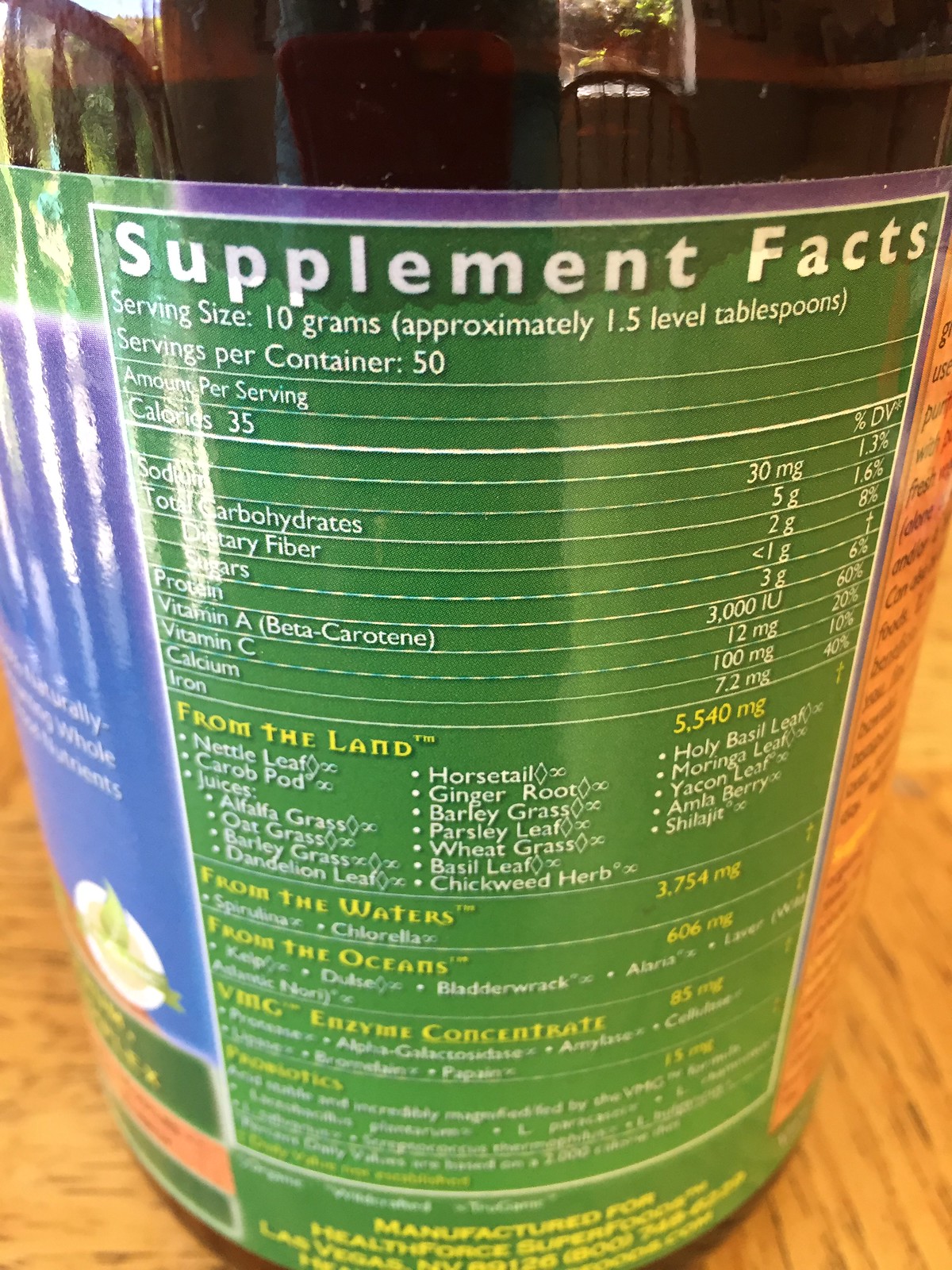This image features a detailed supplement facts label from a green bottle of vitamins produced by Health Force Superfoods, based in Las Vegas, Nevada. The label is primarily green with white text, with certain headings like "From the Land" and "From the Waters" highlighted in yellow. The serving size is 10 grams, approximately 1.5 level tablespoons, with 50 servings per container. Each serving provides 35 calories, 30 milligrams of sodium, 5 grams of total carbohydrates including 2 grams of dietary fiber and less than 1 gram of sugars, and 3 grams of protein. The supplement is rich in various vitamins and minerals, offering 60% of the daily value for vitamin A (3000 IU of beta-carotene), 20% for vitamin C (12 milligrams), 10% for calcium (100 milligrams), and 40% for iron (7.2 milligrams).

The ingredients are divided into various categories including "From the Land," which encompasses nettle leaf, carob pod, alfalfa grass, oat grass, barley grass, dandelion leaf, horsetail, ginger root, parsley leaf, wheat grass, basil leaf, chickweed herb, holy basil leaf, moringa leaf, yacon leaf, amla berry, and shilajit. There is a notation mentioning concentrates and probiotics, though these specifics are less clear. The overall label design and organized horizontal lines categorize the nutritional information and ingredients meticulously.